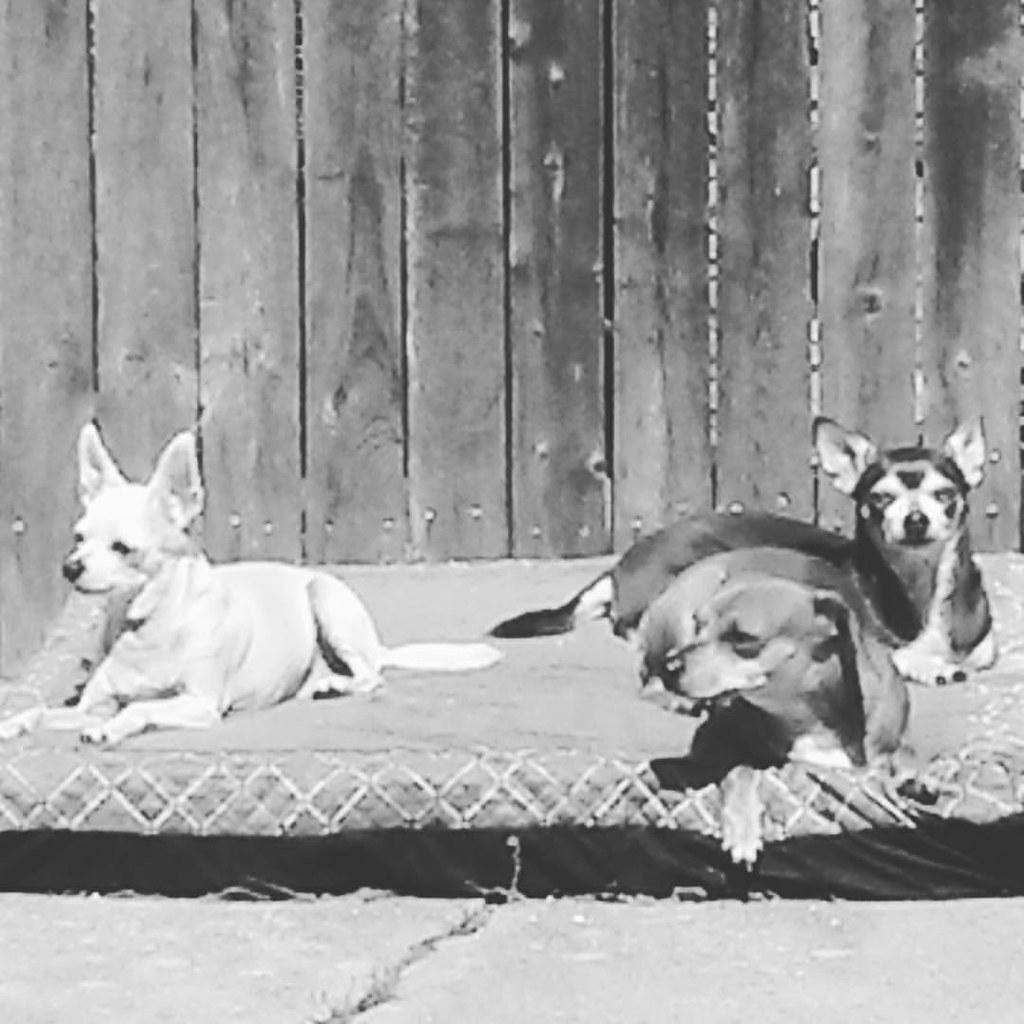This black and white photograph captures a charming scene of three chihuahuas lounging on a rectangular dog bed with a patterned border, set on a concrete or asphalt walkway with a prominent crack running through it, where small weeds and grass are sprouting. The backdrop consists of vertical wooden planks with two visible nail holes at the bottom of each board, forming a rustic fence. The chihuahuas are arranged with a tan or light-colored one on the left, which is lying down and looking off to the left side of the photo. Next to it, towards the right, is a darker chihuahua, also gazing to the left, appearing relaxed with drooping ears. Behind them is a black chihuahua with a light-colored face and a distinct dot on its forehead. This dog is looking directly at the camera with an almost displeased expression. The sunlight highlighting the scene adds to the peaceful outdoor setting, adding depth and texture to the various elements within the image.